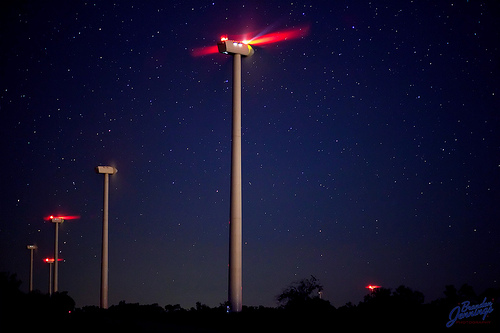This atmospheric photograph, possibly computer-generated, captures a stunningly detailed night sky filled with numerous faint white stars against a gradient that transitions from deep black at the top to dark indigo and lighter blues near the horizon. The image features a row of five tall, slender lampposts, each with T-shaped horizontal light fixtures at the top. These lampposts, which are a pale brown or tannish color, recede into the background, emphasizing their perspective and height above a faint tree line at the base of the image.

The lampposts are striking in their appearance, with the foremost pole dominating the center of the frame. The lights atop these poles emit a vivid reddish-orange glow, with hints of yellow. However, not all lights are lit; the second and the fifth poles from the left do not have illuminated lights, creating an intriguing pattern of light and shadow. The absence of light on these poles contrasts sharply with the bright bursts from the others.

Adding to the artistic detail, there is a signature in blue script, likely reading "Brandon Jennings," located in the lower right-hand corner, confirming a touch of personal craftsmanship in the piece. The combined elements of the star-speckled sky, the towering lampposts, and the subtle treeline create a mysterious yet captivating scene that leaves one pondering its realism and the purpose of its luminous towers.